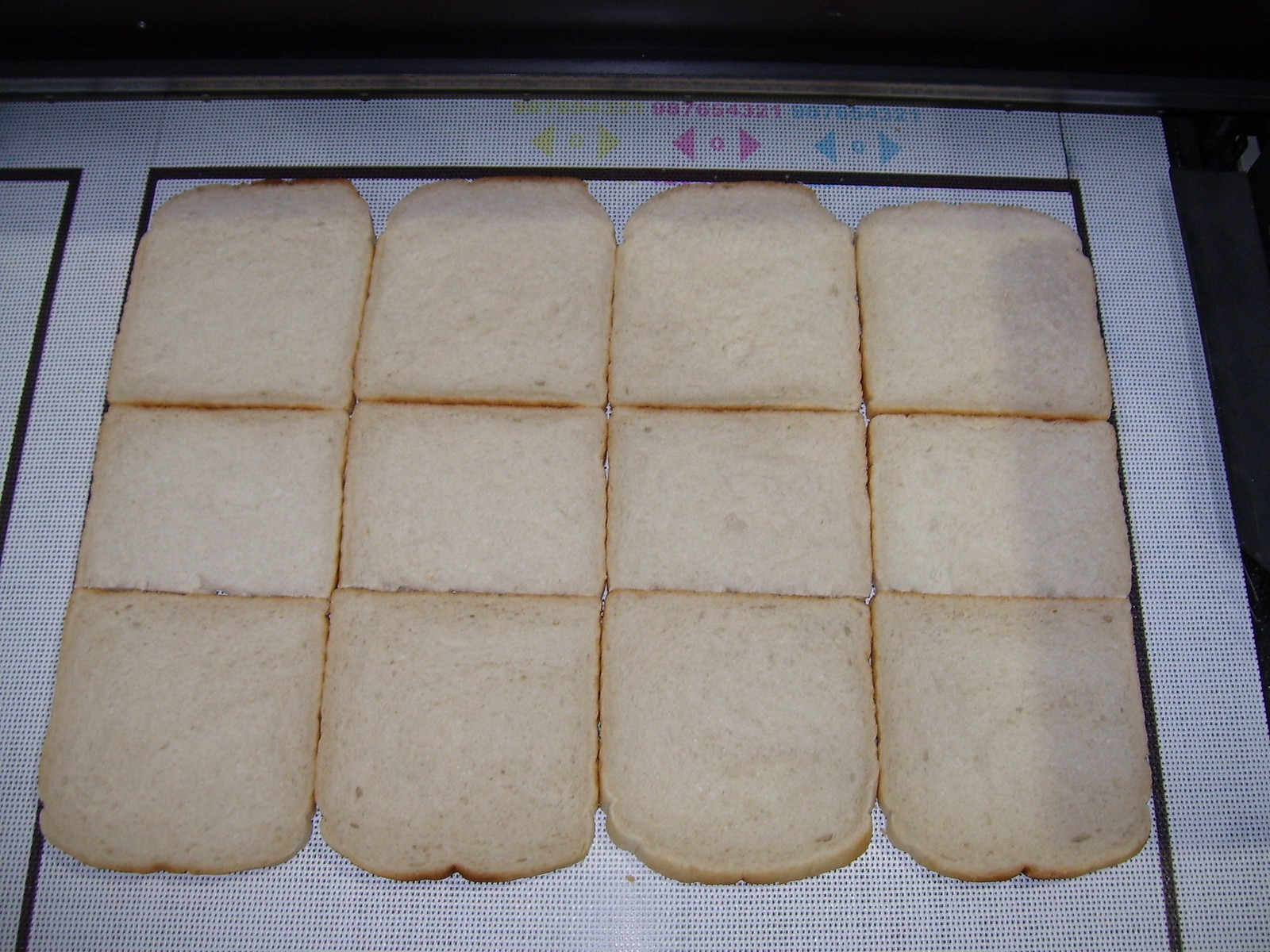This is a detailed color photograph likely depicting a computer or LCD screen. The image has a black border with text at the top that is difficult to read, featuring yellow, pink, and blue arrows pointing left and right. The screen itself is primarily gray and outlined in a black square. Within this square, there are twelve slices of white bread arranged neatly in three horizontal rows of four slices each, touching side by side. The bread slices are light white-yellowish in color, with rounded tops and bottoms while the middle section remains straight. The overall layout of the bread suggests a band-aid shape pattern, and just noticeable toward the left is the outline of another black square. At the bottom of the image, a light gray paper or placemat with black lines forms the base of the display.